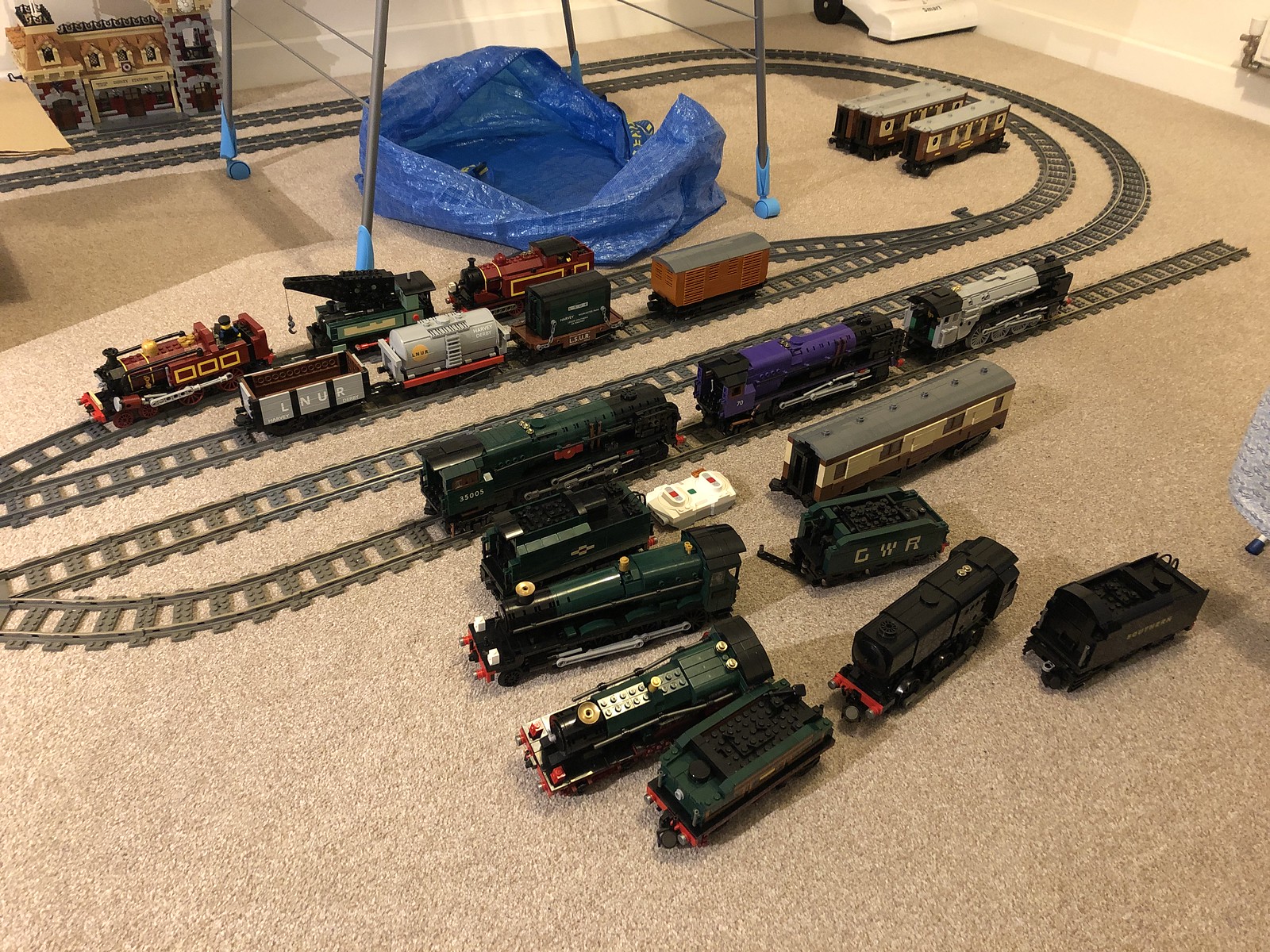The photo depicts an elaborate model train set arranged on a brown, pile carpet in an indoor room. The centerpiece is a table with four steel legs that have blue wheels, and beneath it lies a blue tarp. Surrounding the table, an extensive train track network extends across the floor, threading through ceramic tiles in the background. Scattered around the tracks are various train cars in an array of colors, including red, gray, yellow, green, black, tan, and an orangish brick hue. Notably, about half of these train cars rest on the carpet rather than on the tracks, indicating a bustling and possibly in-progress setup. In the upper left corner of the image, a miniature train station adds a touch of realism, while a vacuum cleaner is visible in the upper right corner. Additional elements include remote controls and a blue bag positioned opposite the train tracks, suggesting that the model train setup is a dedicated hobby space.